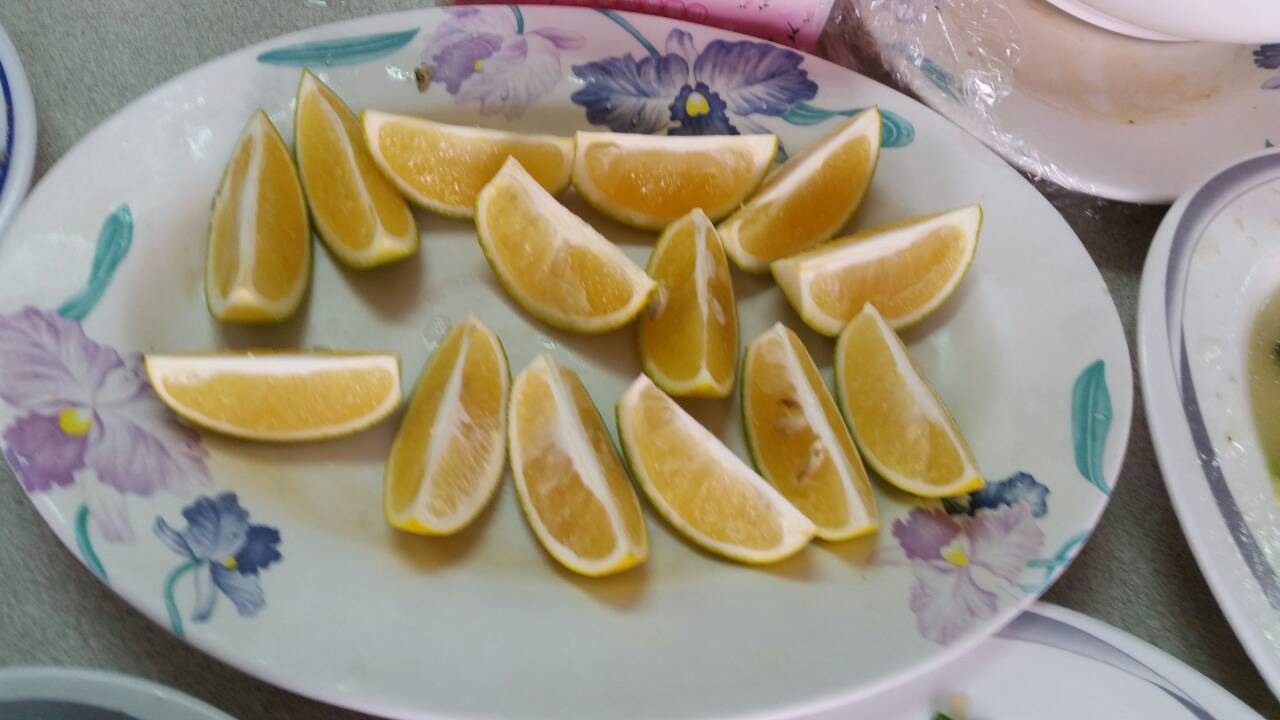The photograph, taken in a landscape orientation, captures a central white plate adorned with beautiful blue and purple floral patterns, featuring turquoise stems and leaves. The plate, viewed from a 45-degree angle above, is slightly concave with a higher outer lip. At its center, laid rind-down and flesh-up, are 10 to 12 wedges of brightly colored citrus fruit, possibly lemons or oranges, some of which reveal seeds or pips. Surrounding this main plate are several other plates on a light grayish table, though their contents are mostly obscured, revealing only hints of food residue and decorative patterns, including a plate with a blue and white line around its edges. The light indoor setting and the meticulous arrangement of the fruit and plates create a pleasing and detailed still-life composition.